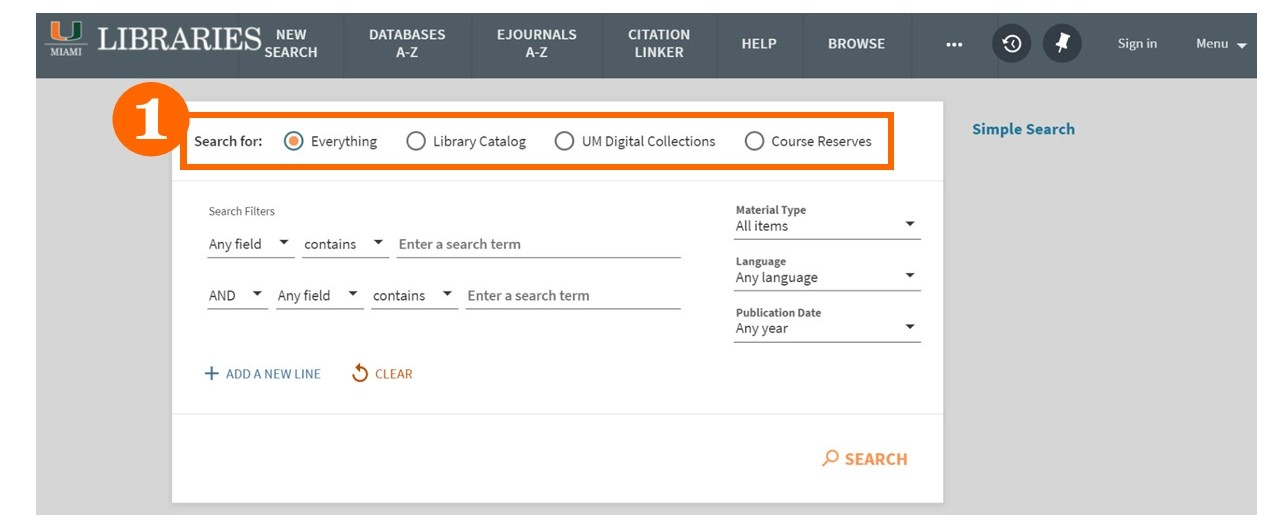Screenshot of the University of Miami Libraries Search Page

This image displays a screenshot of the University of Miami Libraries search interface. The page has a clean, light gray background with a darker gray border at the top. Prominently featured at the top is the University of Miami’s emblem in the institution’s signature orange and green colors, accompanied by the text “Miami” in a very small font below the emblem. To the right, the word “Libraries” is displayed in all caps with a large white font.

Below this header, there are several navigational links: “New Search,” “Databases A-Z,” “E-Journals A-Z,” “Citation Linker,” “Help,” and “Browse,” each clickable individually. Additionally, there is a three-dot menu icon (often referred to as a hamburger menu), a "Recents" button, a "Pin" button resembling a push pin, a "Sign In" button, and a drop-down menu button.

Encapsulated in an orange rectangle with a large orange circle containing the number "1" in white text, there is a search bar with the prompt “Search For,” indicating the user has selected the “Everything” option. Below the search bar, there are search filter options where users can add new lines, clear filters, and specify criteria such as material types, language, and publication date. The search button, highlighted at the bottom right, finalizes the search once the user has entered their specific filter parameters.